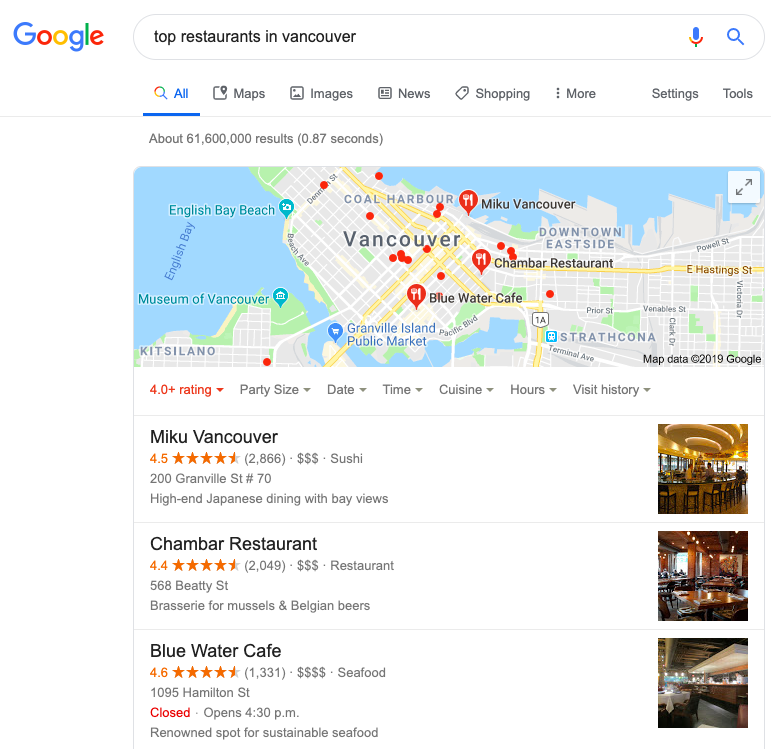The image displays a Google search results page for "top restaurants in Vancouver." On the top left, the familiar Google logo is visible. The search query has returned a map with multiple pin locations indicating various dining options within Vancouver. Detailed below the map are listings of several top-rated restaurants.

1. **Mike Vancouver** - This restaurant boasts a rating of 4.5 stars. Located at 200 Craneville Street, the establishment is described as offering high-end Japanese dining with beautiful bay views.

2. **Chamber Restaurant** - With a 4.4-star rating, this restaurant is situated at 568 Beattie Street. It is noted for its brasserie setting, specializing in mussels and Belgian beers.

3. **Blue Water Cafe** - This spot holds an impressive rating of 4.6 stars and can be found at 1095 Hamilton. It is currently marked as closed but will reopen at 4:30 p.m. The restaurant is renowned for its sustainable seafood offerings.

This comprehensive depiction provides a clear and informative guide for anyone looking to explore some of Vancouver's top dining establishments.